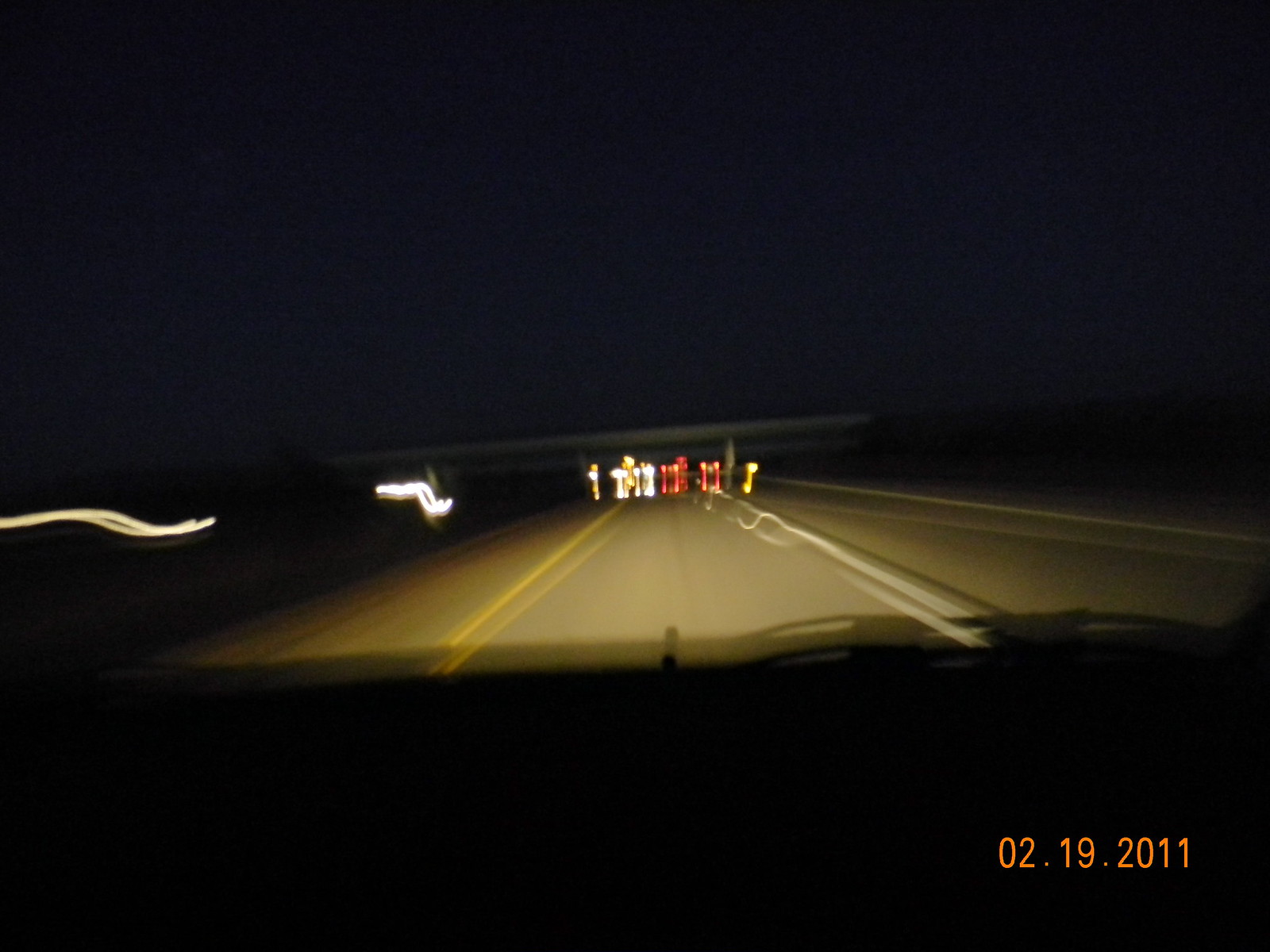This image captures a blurry nighttime view from a moving car, likely from a dash cam. The pitch-black sky reveals no stars or trees, emphasizing the darkness of the scene. The car is traveling down a highway, with visible white lines marking the lanes and a double yellow line in the center. On the left side, lights from oncoming traffic illuminate the road. A bridge is visible ahead, and in the distance, there are numerous poles, possibly part of a construction area, with red, yellow, and white colors, some with lights. The bottom right corner of the image has an orange timestamp reading "02-19-2011," signifying the date it was taken.